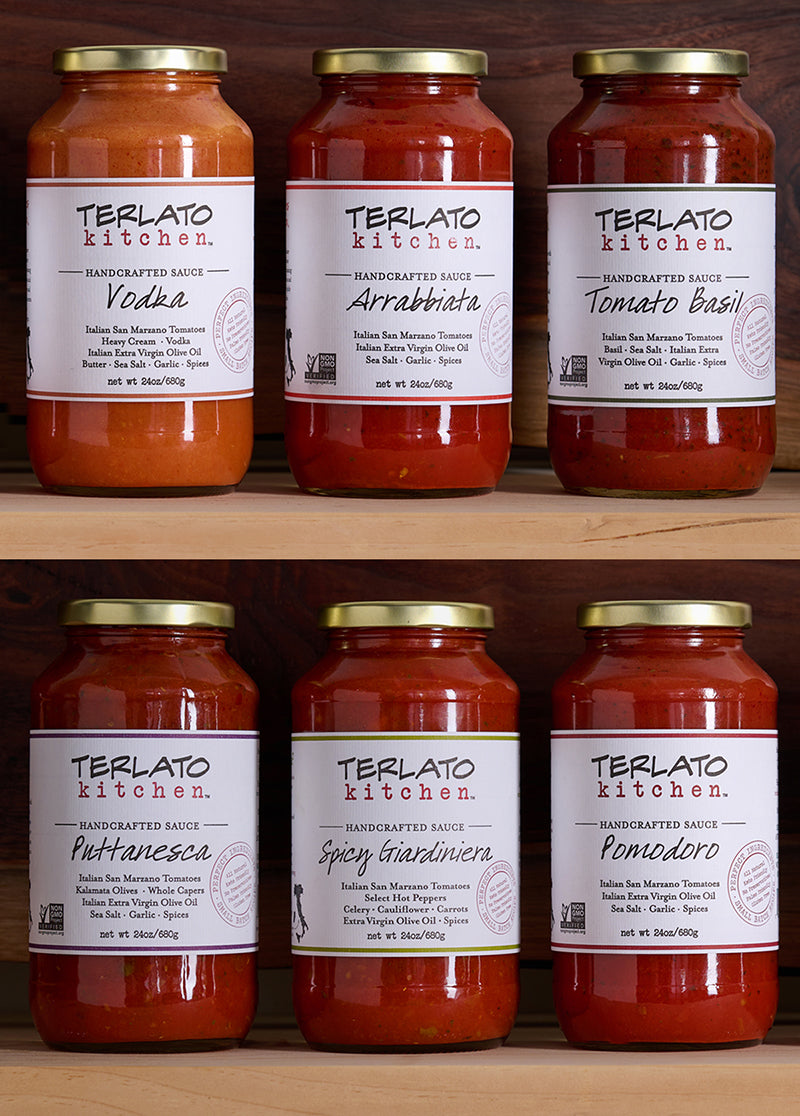This is a vertically aligned rectangular image depicting six jars of pasta sauces arranged on two light brown wooden shelves within a cabinet-like structure. Each jar is capped with a gold lid and features a white label from the brand Terlato Kitchen, inscribed with black lettering. On the top shelf, from left to right, the sauces are: Vodka Sauce, which is notably more orange in color; Arrabbiata Sauce, a vibrant red; and Tomato Basil Sauce, a darker red hue. The bottom shelf houses three uniformly dark red sauces: Puttanesca Sauce on the left, Spicy Giardiniera Sauce in the middle, and Pomodoro Sauce on the right.